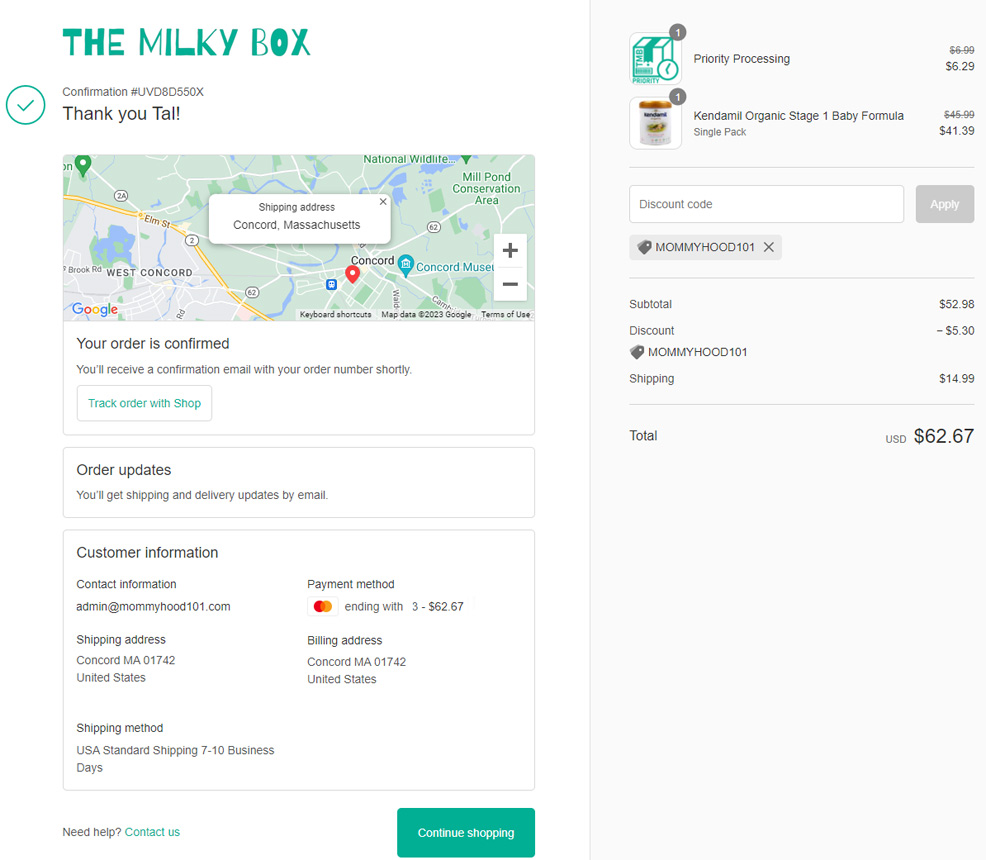The image depicts a checkout confirmation page from an online shopping site. The familiar layout suggests it's part of an e-commerce platform. 

In the upper left-hand corner, there’s a logo labeled "Milky Box" in green. There is text indicating the confirmation of an order, but it’s too small to read clearly. Below the confirmation text, there’s a message saying "Thank you, Tia." 

Further down, there’s a section showing the shipping address accompanied by a map indicating the location in Concord, Massachusetts. The order confirmation statement reassures that a confirmation email with the order number will be sent shortly. There’s also an option to track the order using the "Shop" feature for order updates.

The "Customer Information" section is displayed next, including contact information (admin@nomihood131.com), shipping address, billing address, and the payment method, which appears to be a MasterCard ending in 6237. The shipping method is noted as "USA Standard," with an estimated delivery time of 7-10 business days. A "Need Help? Contact Us" link is provided, along with a green "Continue Shopping" button.

On the right-hand side of the page, the items included in the order are detailed:
1. **Priority Processing** priced at $6.29, reduced from a higher price that is crossed out.
2. **Candrani Organic Stage 1 Baby Formula** – there’s a picture of the baby formula tube, priced at $41.09, reduced from $44.19.

Below the items, a discount code is applied (potentially "Mommy HO22101" or "HOD101" though it is hard to decipher). The subtotal is displayed as $52.98, with a discount of $6.30. The shipping cost is $14.99, bringing the total to approximately $62.67 or possibly $82, as the small text makes it difficult to ascertain the exact figure.